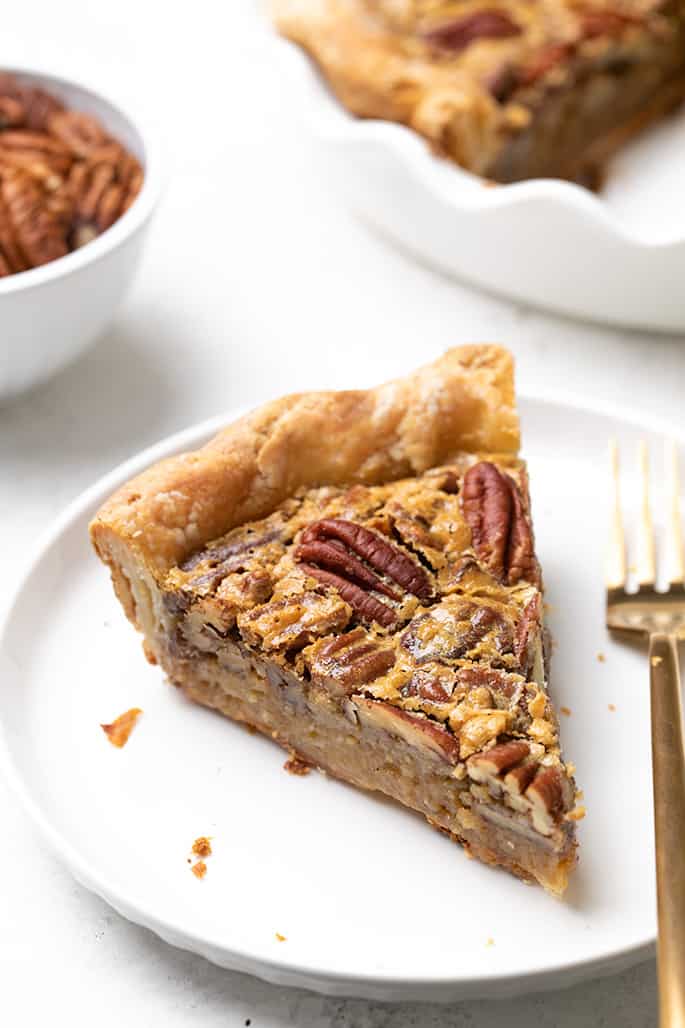In this food magazine-worthy photograph, set against a plain white background, a tantalizing slice of pecan pie takes center stage on a pristine white round plate. A few crumbs from the flaky, golden crust pepper the plate, adding a touch of rustic charm. A gold fork lies elegantly beside the slice, inviting a taste. Behind this, slightly out of focus but still discernible, sits a portion of a matching white pie dish with an undulating edge, showcasing the rest of the pie from which the slice was taken. To the left, a white bowl filled with pecans – presumably the key ingredients of the pie – adds a complementary detail. The simplicity of the white background and tablecloth accentuates the rich tan and dark brown hues of the pecan pie, highlighting its textured layers: the crunchy pecan topping, gooey filling, and its perfectly baked crust. The composition and color scheme of the photograph intimately celebrate the allure and intricacies of this classic dessert.